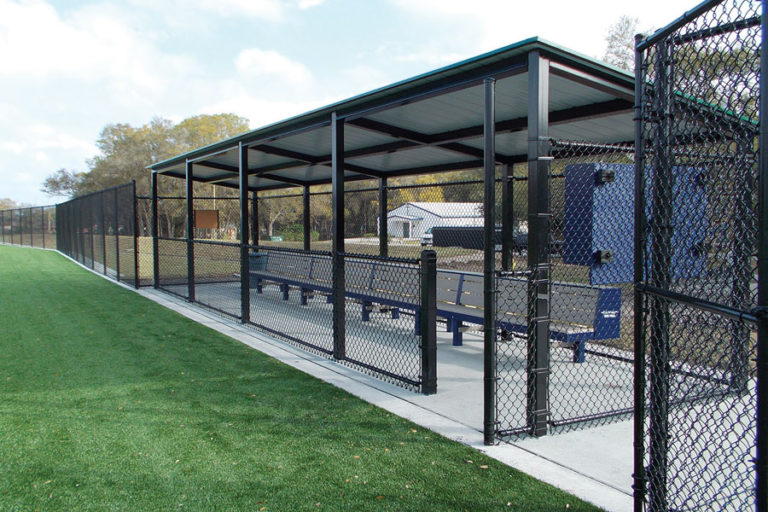The photo captures a segment of a large, green grassy field with black fences stretching as far as the eye can see. In the foreground, a fenced-off seating area with a slanted cover is visible, featuring a single row of blue benches with white legs situated on a white stone base. To the right of this seating area, the ground transitions to yellowing grass. A one-story, white building with a triangular roof is present in the background, surrounded by numerous trees. The scene also includes a brown sign near the left side of the fence, which borders the grassy field. Additionally, there are openings in the fencing, suggesting pathways leading onto the field. Overall, the setting conveys a designated rest or lookout area, likely intended for observing activities on the field.